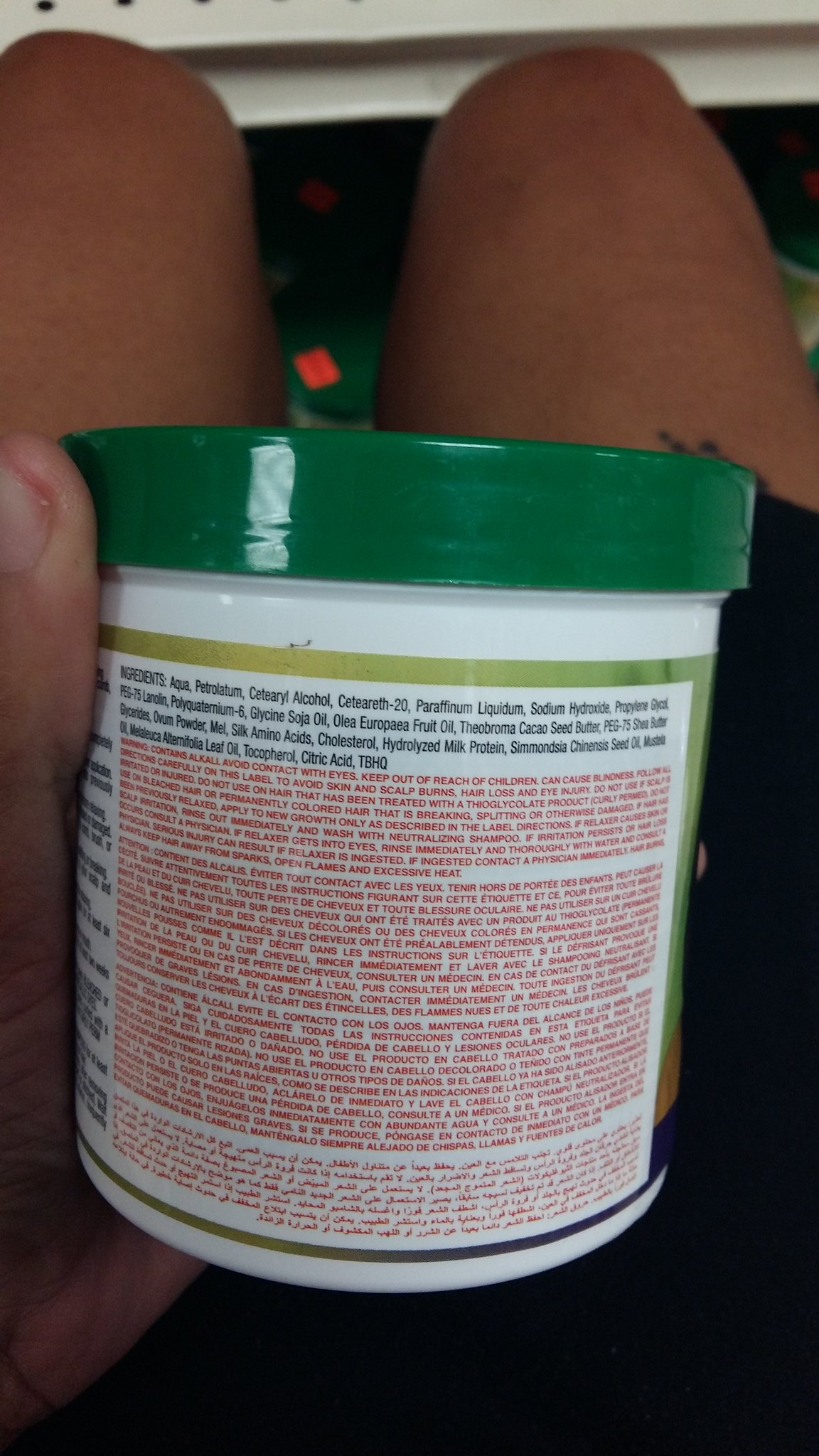In this portrait-oriented photograph, the focal point is a green plastic canister with a matching green lid, prominently displayed in the center. The canister is held by a human hand, with the thumb clearly visible along its side. The jar is shown with its back label facing the camera, adorned in a gold rim with small red font text that covers much of its surface. Black writing is also noticeable near the top of the lid. The jar is held by a person who appears to be female, wearing a black dress. Her Caucasian knees are visible at the top of the photograph, indicating she is in a seated position. The background features dark flooring with a red diamond pattern, while the carpet in front of her is green, also patterned with red diamonds.